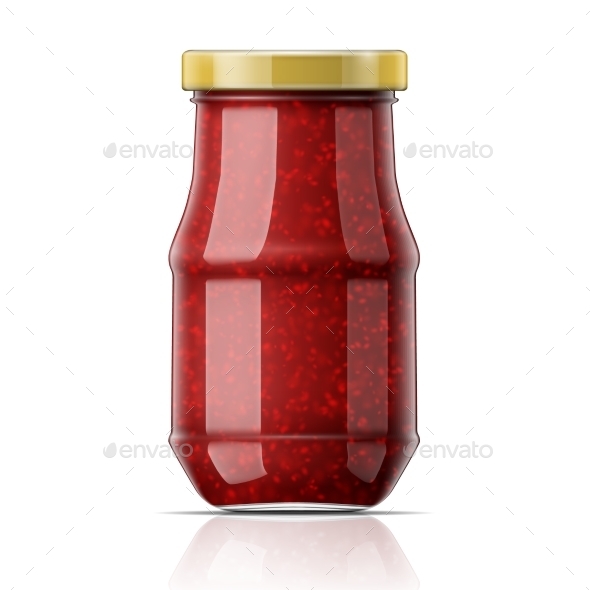The image depicts a centrally positioned glass jar filled with bright red sauce or jam, characterized by an abundance of white seeds. The jar prominently takes up almost the entire frame, set against a clean, fully white background. The jar features a yellowish lid and is marked by four watermarks that read "Envato," which likely indicates the brand or company associated with the image. The colors within the photo include vivid red, white, gray, gold, and black. The image bears the traits of stock photography, potentially sourced from a clipart or stock image website, possibly for commercial use by Envato. The overall setting and style unequivocally suggest that the image is used as a product representation, emphasizing the detailed depiction of the jar and its contents.